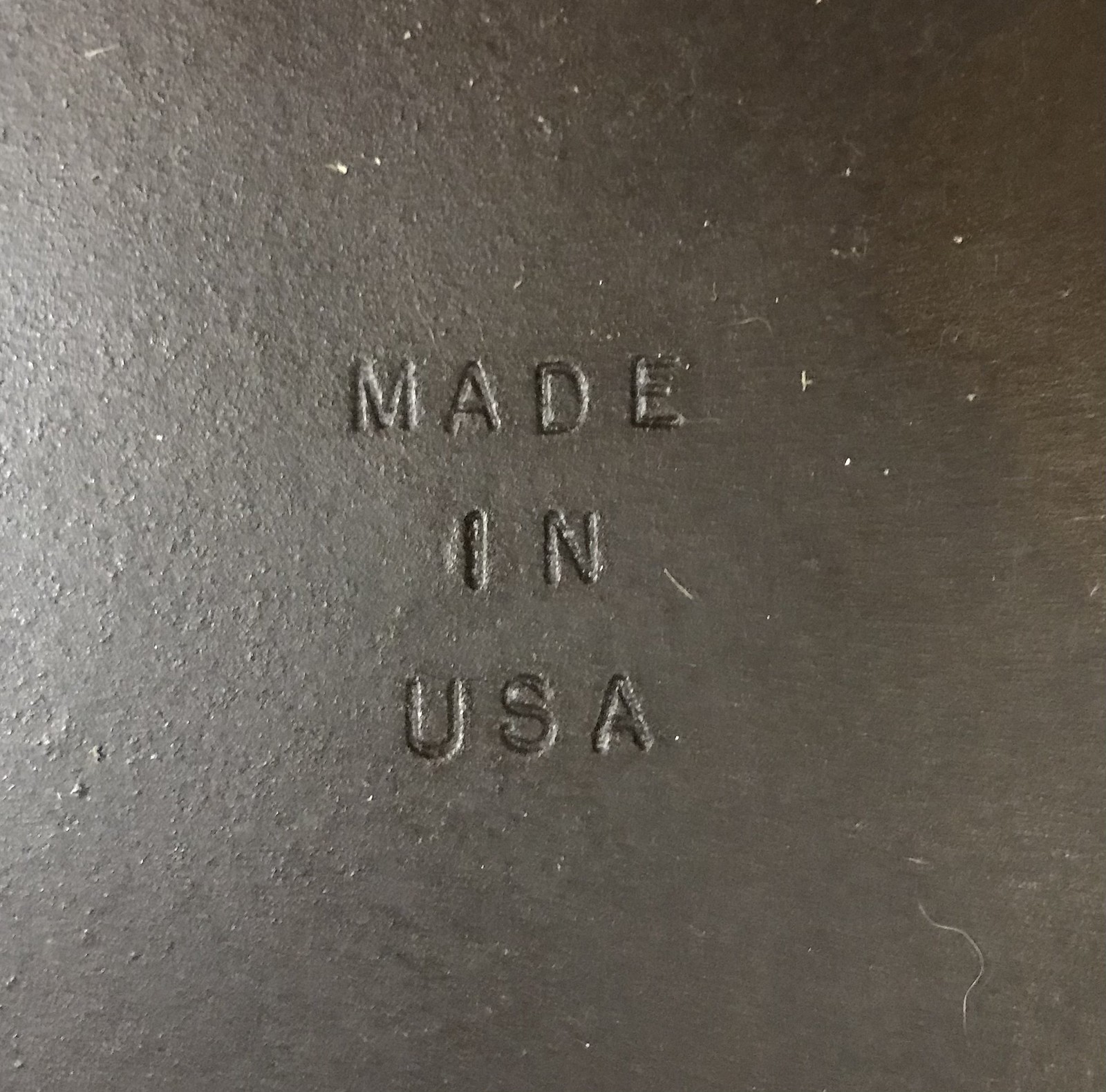A close-up photograph captures a rugged slab of iron with noticeable granularity, indicating it has not been finely processed. The surface displays various imperfections, including a stray body hair and patches of lighter-colored dirt. The phrase "Made in USA" is prominently imprinted on the metal, instilling a sense of pride in its origin. The iron piece occupies the entire frame, leaving no background visible. Lighting from the left side of the image highlights the texture and unevenness of the metal, emphasizing its raw and industrial nature.